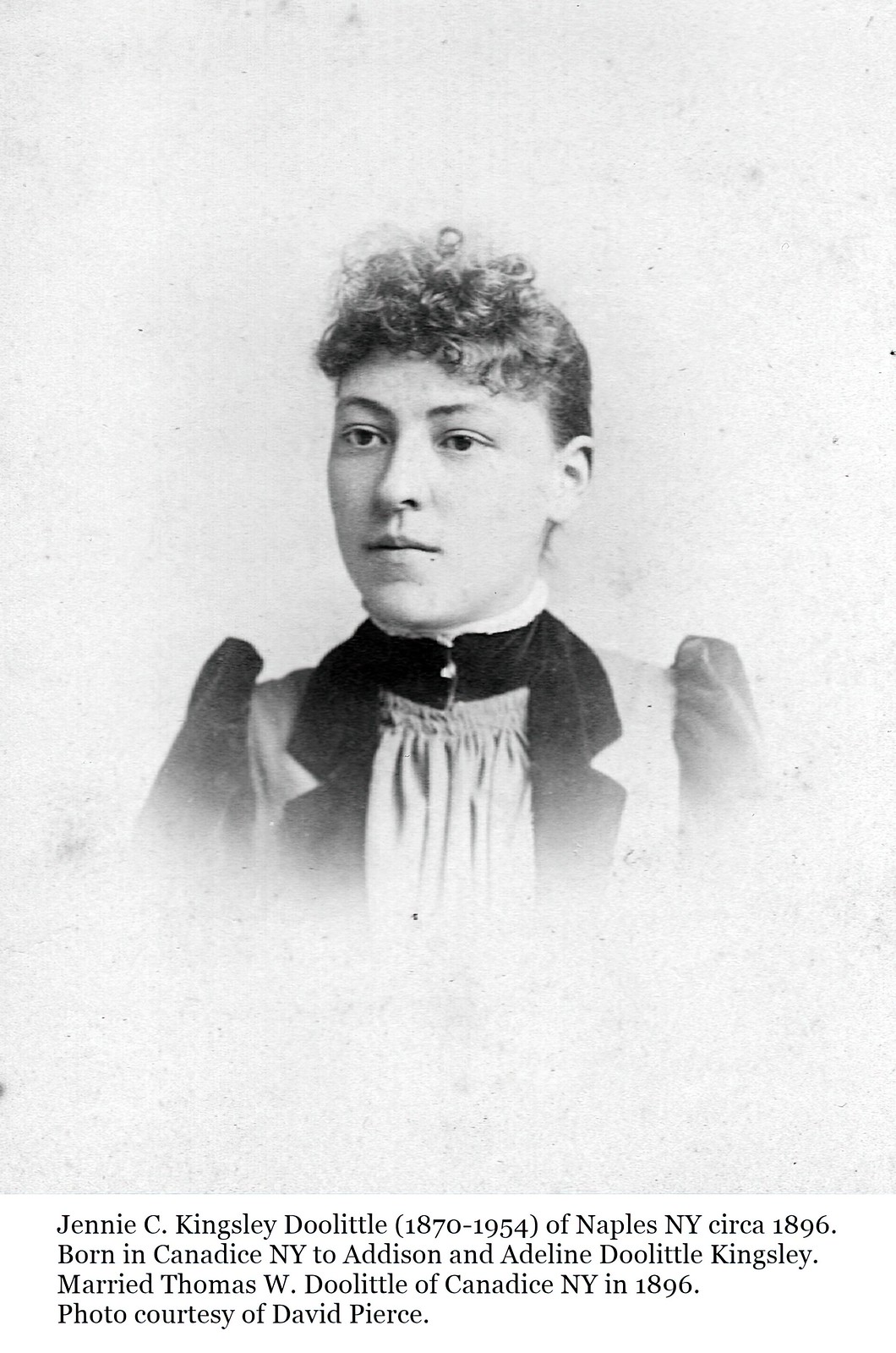This detailed black-and-white photograph, showcasing a woman from the late 1800s, is centered on Jenny C. Kingsley Doolittle. She is depicted with curly hair styled in the front and pulled back, wearing a dress characterized by puffy shoulders and a high collared neck with a button at the center. Her neutral expression complements the plain white background that fades out around the chest area, emphasizing the aged nature of the photograph. The text beneath the image reads: "Jenny C. Kingsley Doolittle, 1870 to 1954, of Naples, New York, circa 1896. Born in Candace, New York to Addison and Adeline Doolittle Kingsley. Married Thomas W. Doolittle of Candace, New York in 1896." This historical photograph is courtesy of David Pierce, offering a glimpse into the life and time of Jenny C. Kingsley Doolittle.